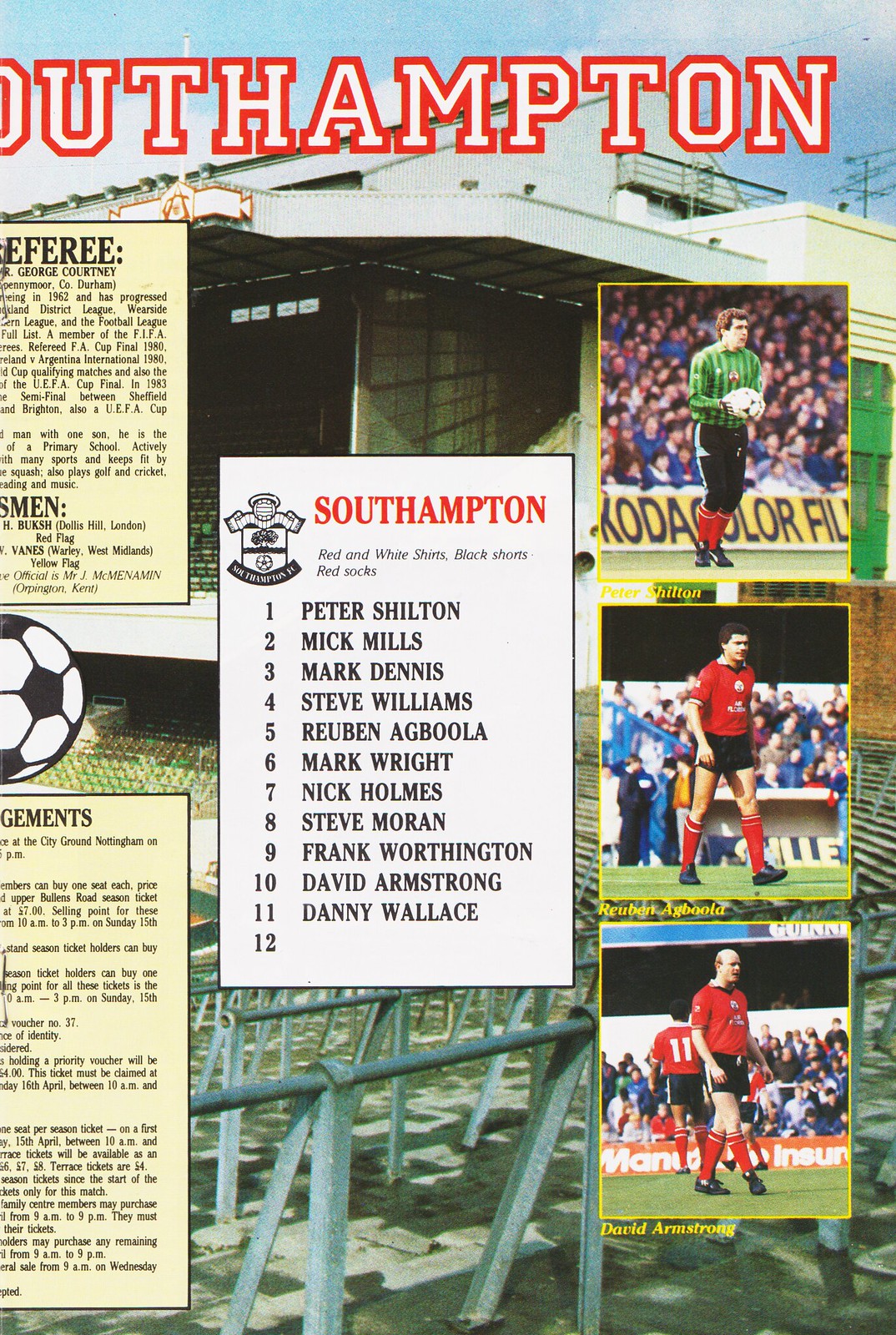This image is of a football program page, likely from Southampton FC, viewed from the right half of a two-page spread. The top of the page displays the word "Southampton," although the "S" and part of the "O" are cut off due to the cropping. The entire background appears to be an inside view of the Southampton stadium. 

The centerpiece is a white rectangle, with "Southampton" in red text at the top. Below this title, the page lists players with red and white shirts, black shorts, and red socks. The team roster includes Peter Shelton, Nick Mills, Mark Dennis, Steve Williams, Reuben Agboola, Mark Wright, Nick Holmes, Steve Moran, Frank Worthington, David Armstrong, and Danny Wallace, numbering from 1 to 12.

Adjacent to the roster on the right, there are three vertically aligned pictures of football players bordered in yellow. The top image shows a player in a green striped shirt, likely a goalkeeper, holding a soccer ball and wearing black pants and red socks. Behind him, spectators and a blue-lettered banner with a yellow background are visible. The middle picture features Reuben Agboola in a red shirt, black shorts, and red socks. The bottom picture is of David Armstrong, similarly attired in a red shirt but paired with blue shorts. 

On the left side of the roster section, there are multiple blocks of text with varying background shades of cream and white, though much of the content is obscured or cut off due to the image's cropping.